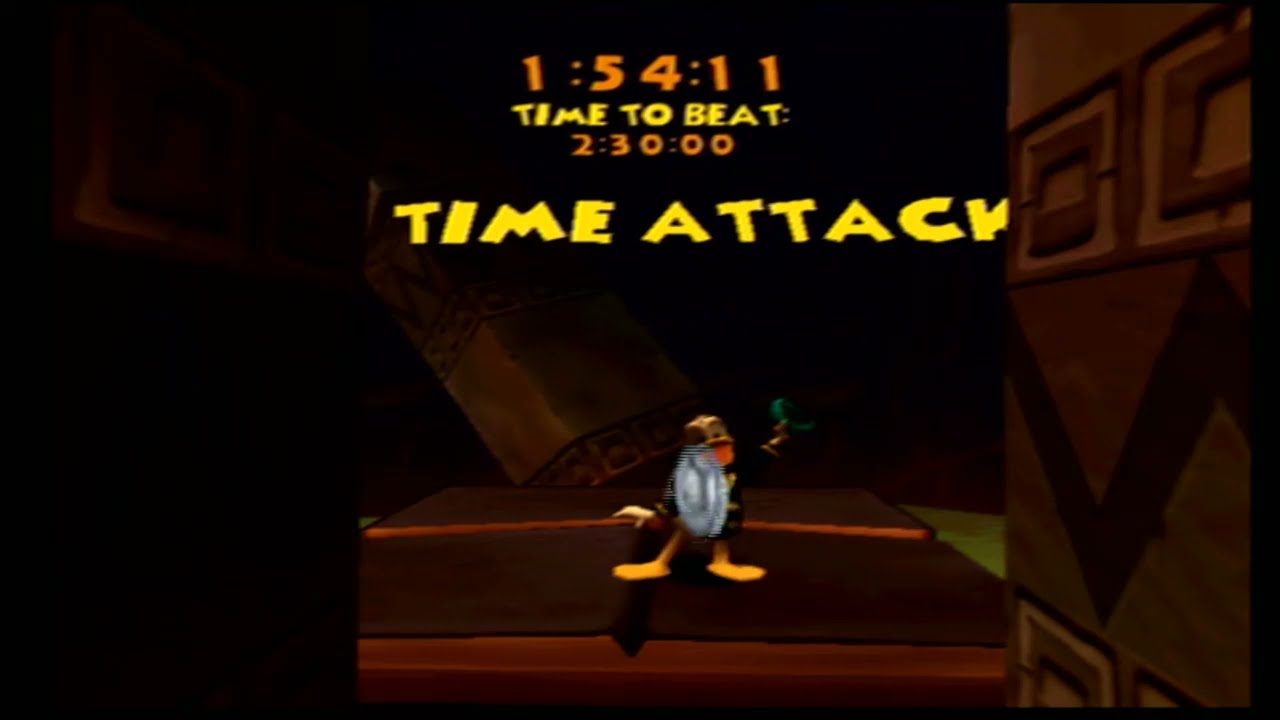The image is a low-quality, highly-pixelated screenshot of a video game, prominently displaying Donald Duck in a miniaturized form. He stands on a platform amidst what could be fallen buildings or books on a bookshelf, obscured slightly by a spherical, chrome-grey graphic. Donald appears animated, with orange webbed feet, his right arm raised holding a greenish-blue object, while his left arm extends back. His tongue sticks out, adding to his animated demeanor. The stage around him is a mix of dark red and brown shades, flanked by a big brown wall on the right, etched with a darker V-shaped design and two squares. On the left side, there's a dark, empty rectangular space. Above Donald, yellow text angled slightly to the left reads "Time Attack," partially cut off by the adjacent wall. Above this, the time 1:54:11 is displayed in orange, with a line of yellow text below reading "Time to Beat," followed by another orange time, 2:30:00. Donald has successfully beaten the required time, as indicated by the text. The overall size of the image is approximately 7 inches across and 5 inches down.